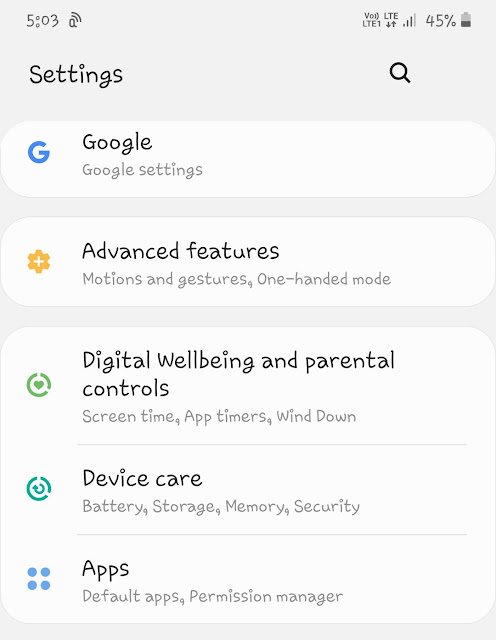A detailed screenshot of an Android mobile device screen displaying its Settings menu. The device uses an unconventional, playful font that deviates from standard serious fonts. The time shown on the screen is 5:03, and the device has three bars of cellular service with a battery level at 45%. At the top right corner, there is a search button for quick access to settings and options.

The visible Settings menu is organized into five distinct categories, each with a corresponding icon on the left and aligned vertically. The categories are as follows:

1. **Google**: Options for Google and Google settings.
2. **Advanced Features**: Includes sub-options for "Motions and gestures" and "One-handed mode."
3. **Digital Wellbeing and Parental Controls**: Contains options for "Screen timer," "App timers," and "Wind down."
4. **Device Care**: Features include "Battery," "Storage," "Memory," and "Security."
5. **Apps**: Encompasses "Default apps" and "Permission manager."

Each category is clearly separated, making it easy for users to navigate through the settings available on their Android device.